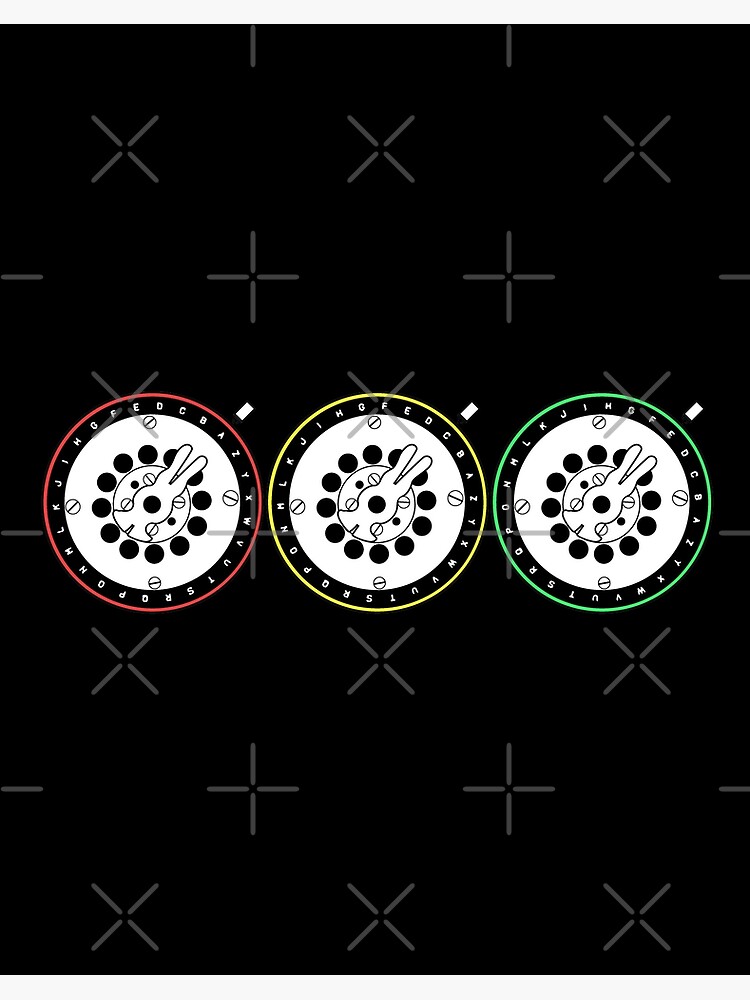The image features a trio of intricate, gear-like watch faces set against a black background. Each watch face is adorned with detailed elements and outlined in distinct colors: red on the left, yellow in the center, and green on the right. The interiors of these watch faces mimic the appearance of old rotary telephone dials, with white centers encircled by black rings that are punctuated with white dots. Towards the outer edge, there is white writing on the perimeters, possibly labeled with the alphabet. Distinctive hand-like shapes extend from the centers, resembling scissors or rabbit ears.

The background is covered in a pattern of alternating gray X's and plus signs, creating a visually engaging backdrop. Intriguingly, the circular watch faces have black holes within them, adding to the mechanical aesthetic. A peculiar clamp in the middle of the left watch face bears a strong resemblance to a bird’s head or a rubber chicken, with its beak forming a peace sign. The symmetrical, side-by-side arrangement of these colorful, detailed circles against the patterned backdrop lends the image both complexity and a striking visual appeal.